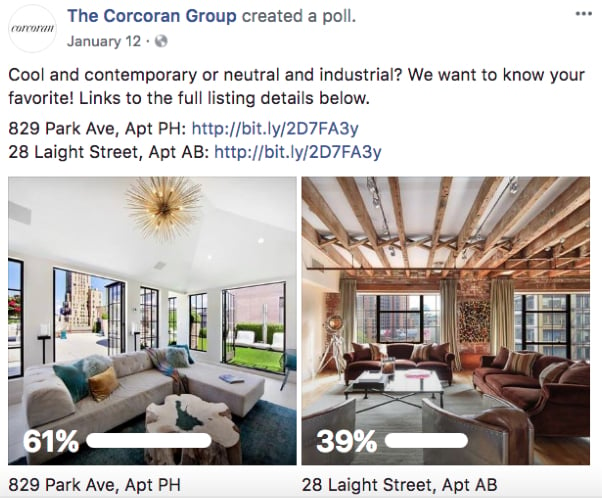In this social media post by the Corcoran Group, the poll invites users to choose between two apartment styles: "Cool and Contemporary" versus "Neutral and Industrial." 

At the top left, the blue text "The Corcoran Group" is prominently displayed. To its right is the text "created a poll." Just below, the question posed is, "Cool and Contemporary or Neutral and Industrial? We want to know your favorite. Links to the full listing details below."

The post then lists two addresses and their accompanying website links: "829 Park Ave, apartment PH" and "28 Late Street, apartment AB." 

Two images of the respective apartments are shown to help users decide. 

The left image, representing 829 Park Ave, features a cool and contemporary design with a light gray color scheme. The room includes a light gray sofa, gray walls, and a gray ceiling. Several windows and doors are partly open, providing a view of natural light. A blue rug adorns the floor, and a chandelier hangs from the ceiling.

The right image, representing 28 Late Street, depicts a neutral and industrial theme. It showcases hardwood brown flooring, brown couches, and a distinctive wooden ceiling made of 6x6 beams, spaced about a foot apart.

At the bottom of the poll, the current standings show 39% favoring the Late Street apartment and 61% favoring the Park Ave apartment.